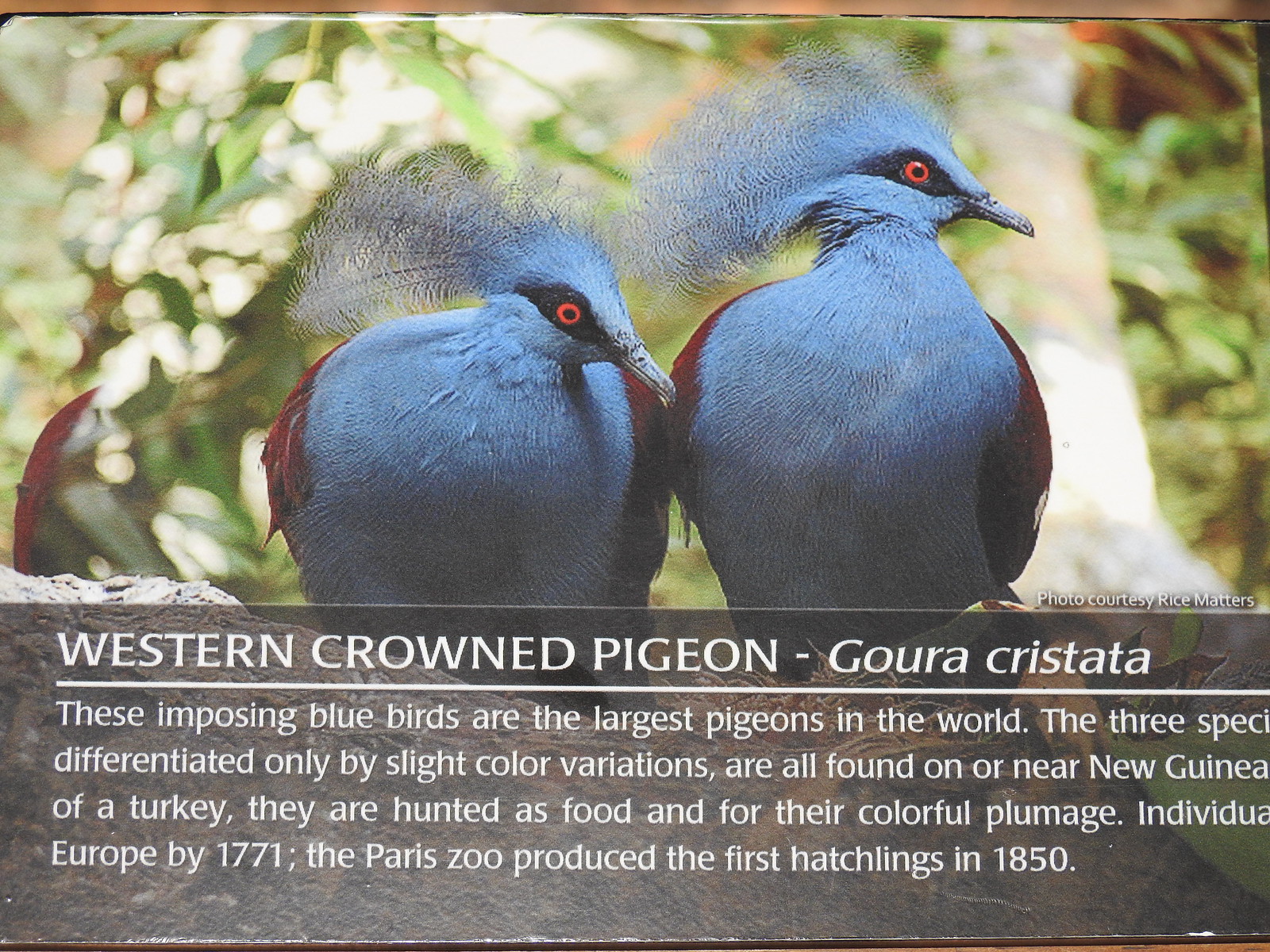This image features two Western crowned pigeons (Gura Christata), distinguished as the largest pigeons in the world. With their striking, light blue, round bodies and bright red eyes, these imposing birds stand side by side, their heads slightly turned to the right. The prominent fuzzy feathers on top of their heads and bluish-gray beaks add to their distinct appearance. Their impressive plumage and red wings make them highly noticeable, and they are often hunted for food and their colorful feathers. The background, slightly out of focus, hints at trees and foliage, suggesting a natural habitat near New Guinea where these birds are typically found. The text beneath the birds provides additional details, mentioning their introduction to Europe by 1771 and their first hatchings at the Paris Zoo in 1850.